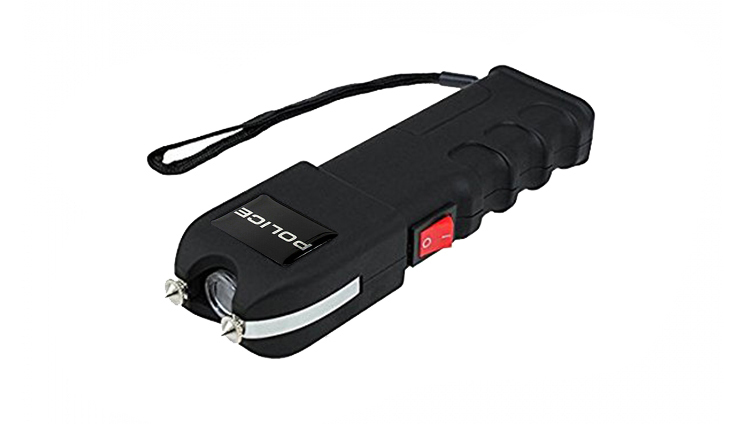The image features a black police taser laying horizontally on a white background. The taser, with its rectangular shape, faces towards the bottom left. At the front end, two sharp, silver-looking prongs or spikes stick out, with a transparent glass-like surface situated between them. Above these prongs, a white line runs up and rightwards, almost touching a red on/off switch located on the right side. This switch, marked with a circle and a dash, is positioned above the finger grips on the handle. The handle itself is equipped with spots for gripping and features a black strap hanging off it towards the left, ending in a circular loop. On the side of the taser is a black square bearing the word "POLICE" in white text, written upside down when viewed from this orientation. The top right back of the taser appears completely flat.